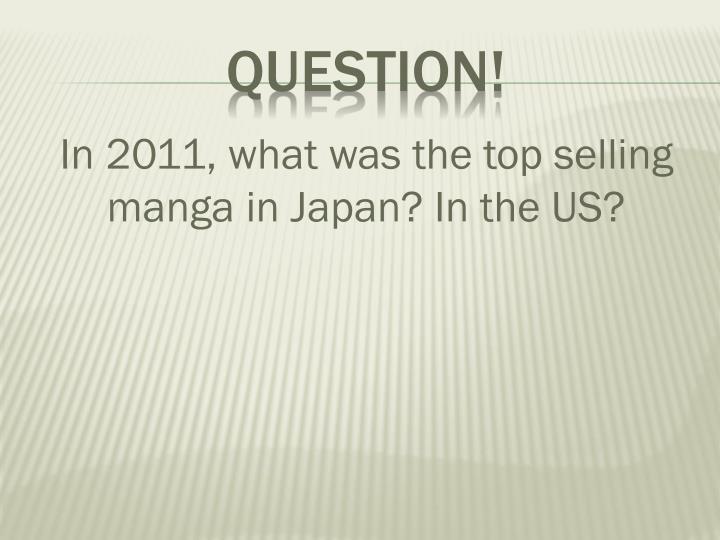The image resembles a PowerPoint slide featuring an off-white, eggshell-colored background with vertical lines, giving a subtle visual texture. At the top center, the word "QUESTION!" is prominently displayed in bold, dark grey letters, with a thin, light blue line running through the bottom portion of the text, creating a reflection effect. Beneath this title, in centered black text, is the inquiry: "In 2021, what was the top-selling manga in Japan? In the US?" The overall background is composed of slightly darker vertical lines against the off-white, adding depth, and at the very bottom, a shadow effect loops around to the side, enhancing the overall dimensionality of the image.